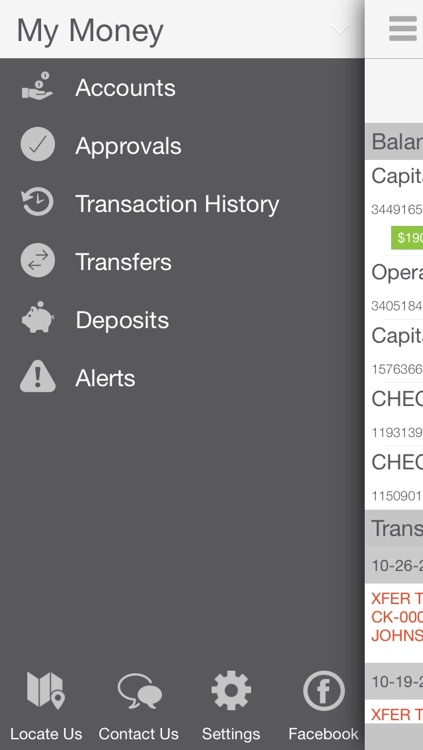This is an image of a mobile banking app interface. The vertical rectangular display starts with a white section at the top that transitions to gray along the right edge. Within this white area, "My Money" is written in gray lettering. Below, the background shifts to solid gray with white text introducing several labeled sections, each accompanied by a distinct icon.

- "Accounts" is marked by an icon resembling a hand holding two balls. 
- "Approvals" features a circle with a checkmark. 
- "Transaction History" is symbolized by a clock with an arrow curving counterclockwise. 
- "Transfers" is indicated by a filled-in circle with arrows pointing left and right. 
- "Deposits" has a piggy bank icon. 
- "Alerts" is represented by a triangle with an exclamation point inside.

Towards the bottom of this section, additional options are available:
- "Locate Us" with a map icon.
- "Contact Us" with two speech bubbles.
- "Settings" featuring a gear wheel.
- "Facebook" shown with a lowercase "f" inside a circle.

To the right of this main section, a sliver of another page is visible, characterized by a white background with three horizontal gray lines at the top. Below, separated by a thin gray line, various text elements are highlighted in gray. 

- The text begins with "B-A-L-A-R."
- Further down, "trans," followed by the date "10-26."
- Even lower is another date, "10-19."
- There is red text at the bottom accompanied by a green box.

After "B-A-L-A-R," regular black text reads "cap" followed by a number, and within a green horizontal box, "$1.19" is partially visible, suggesting an amount or a balance, though the text is cut off.

This detailed caption captures the content and layout of the image, providing clarity on each section and icon depicted.